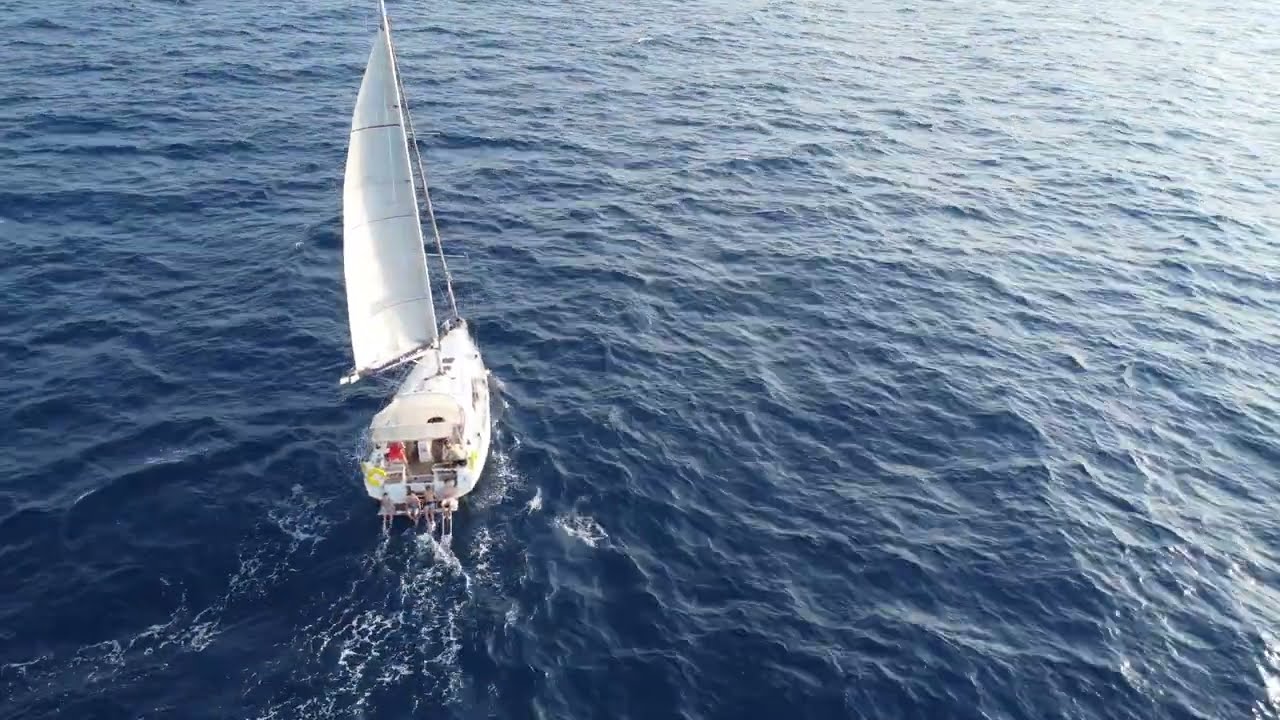In this rectangular image, a white sailboat is sailing on a vast, open body of water. The boat's single, bulging white sail is prominently featured, leaning towards the left with a cable stretching from its top down to the boat. The canopy at the back of the boat shelters several people, including individuals wearing red and yellow. Four shirtless boys in shorts sit at the rear with their legs dangling over the side. The water, a gradient of dark blue to lighter blue and almost white towards the upper right, reflects the sunlight subtly. Behind the boat, ripples can be seen, indicating its forward motion. Additionally, a white speck of light is noticeable in the bottom right, reflecting off the water's surface.